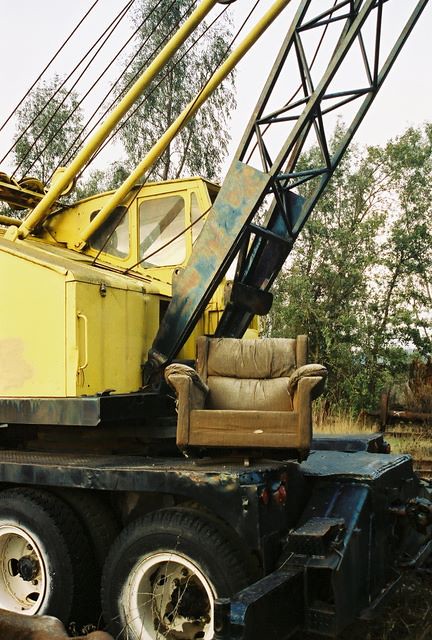The image depicts a worn-out, yellow crane truck with a green telescoping structure extending from its large crew cab, which is situated towards the back of a flatbed platform in a somewhat derelict state. The truck's black rubber tires, each with white rims, rest on the ground, while the platform itself is blue and houses a severely weather-beaten, brown leather recliner with padded cushions. In the background, there is a dense tree line, indicating a green, leafy, wooded area under an overcast, gray sky, suggesting it is daytime.